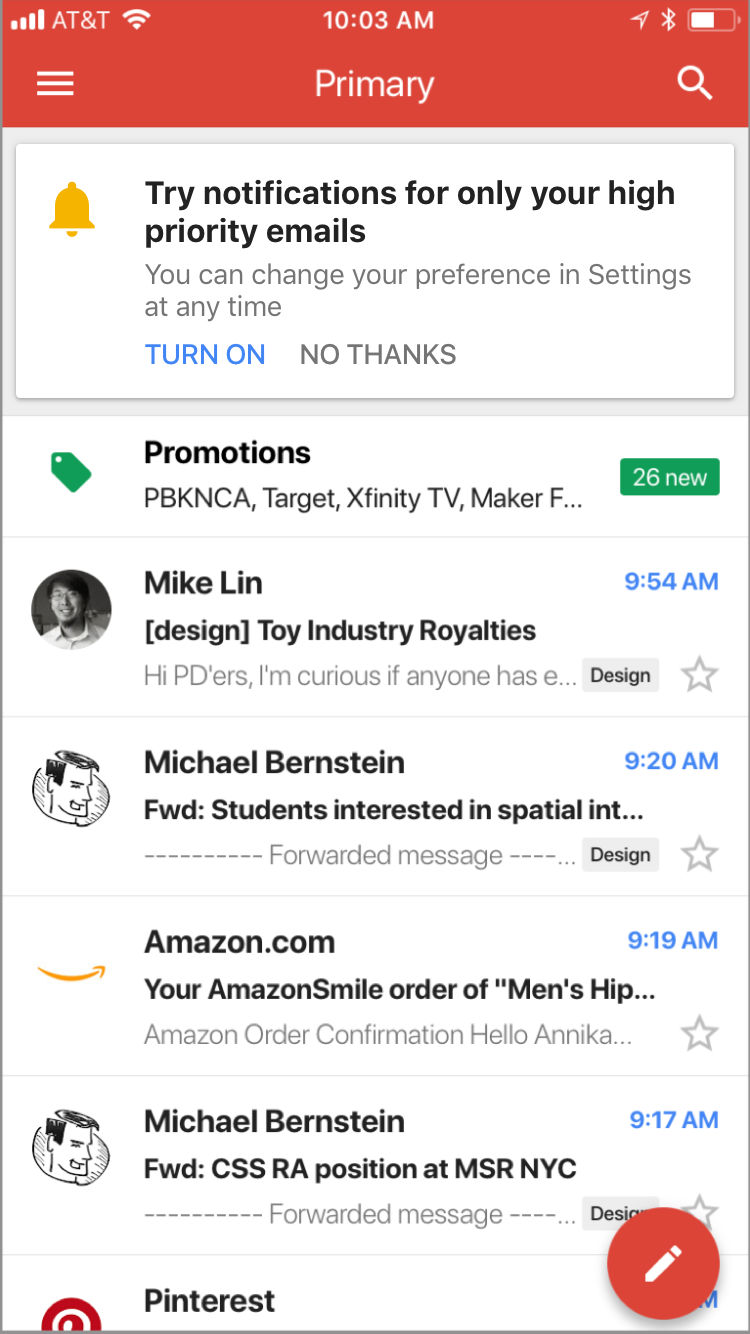The image depicts the Google Mail app on a cell phone, showcasing the primary inbox view. At the top of the screen, a notification banner has appeared, suggesting users try the option to receive notifications exclusively for high-priority emails. The banner reads, "Try notifications for only your high priority emails. You can change your preferences and settings at any time." Accompanying this message are two buttons: "Turn On" and "No Thanks." The high-priority notifications feature allows users to mark certain emails from specific senders as important, ensuring that notifications are received only for these starred emails. This helps in filtering out less relevant notifications, such as spam or newsletters. In the example shown on the screen, no emails are currently marked with a star, including an email from Amazon regarding an order confirmation titled, "Your Amazon Smile order of men's...". If this email were starred, the user would receive notifications for updates from Amazon, highlighting the practicality of the feature.